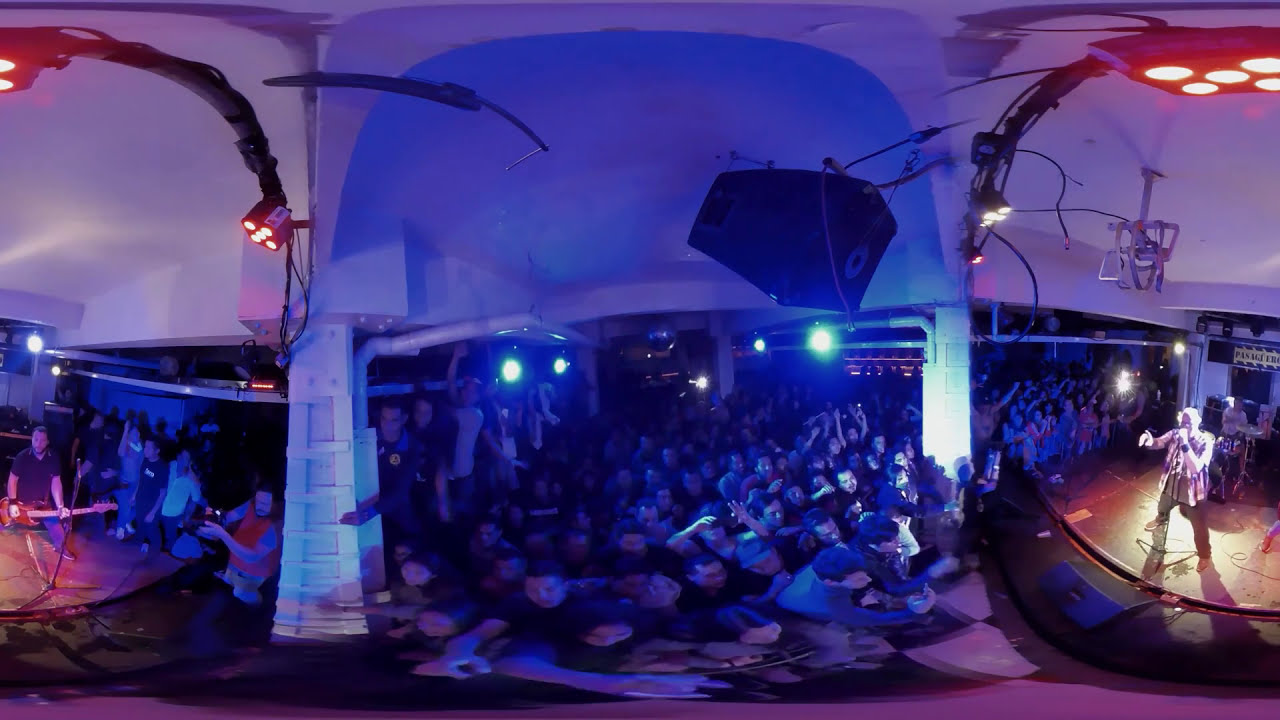This is a horizontally aligned rectangular image, capturing a bustling concert scene though the photograph is quite blurry, especially in the middle area where the majority of the crowd is gathered. The ceiling features black metal arms curved, with red attachments at the end shining multiple spotlights down. The background appears to have white or light gray walls. There's a large group of people densely packed in the center, majority of whom seem to be men, albeit their features are indistinct due to the blur. They have their hands up towards the stage, creating a sea of raised arms. On the left side of the stage, a man in a short-sleeve black shirt and jeans is playing a red guitar. Opposite him on the right side, the lead singer, though blurry, is identifiable by holding a microphone; he appears to be wearing dark pants and has his right arm extended. Above the stage, arched equipment holding the spotlights is visible, contributing to the vibrant and electric atmosphere with colors of red, black, blue, gray, tan, and white reflecting off various elements. The scene seems to be semi-outdoors, possibly at night, adding to the dynamic and immersive ambiance of the concert.